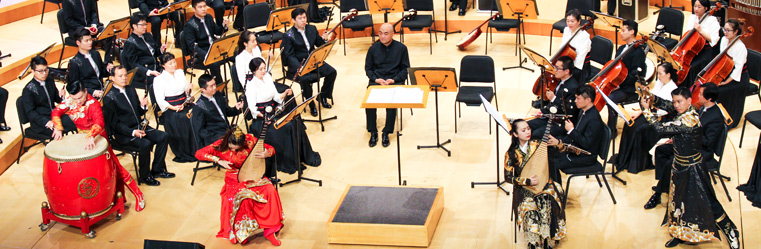The image depicts a wide-angle shot of an Asian orchestra set in a room with a brown floor, lighter colored walls, and wooden beams along the bottom. The seating is tiered, bringing a sense of layered depth to the arrangement. In the foreground, there are two women wearing traditional Asian garb; one plays a guitar-like instrument with a teardrop-shaped body and a long neck, and the other, dressed in a red outfit, also holds a similar instrument. To the left stands a man dressed entirely in red, playing a prominent red Asian-style drum. The background features the rest of the orchestra, with musicians primarily dressed in black skirts and white tops, playing a range of instruments including violins and cellos. In the center sits the conductor, clad in all black with black shoes, positioned behind a podium facing the musicians. A man in traditional attire dances energetically to the right, adding a dynamic element to the scene.